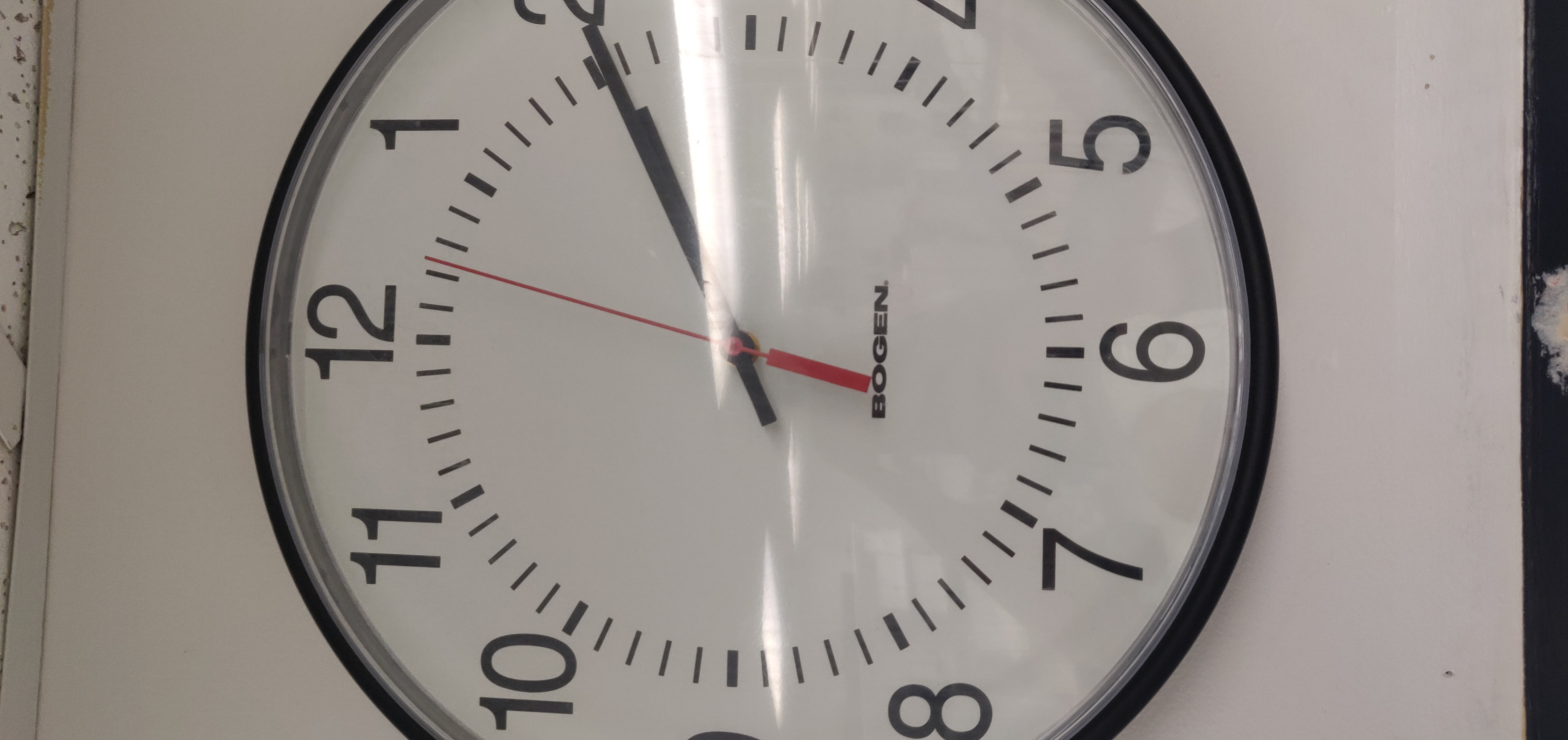The image is a landscape-oriented photograph of a wall clock, turned on its side. The clock's white face is encircled by a black rim, and it has black hour and minute hands, along with a thin red second hand which is positioned approximately two and a half seconds past the 12. The clock shows the time as 2:10. The white clock face features clear black numbers from 1 to 12 and minute increment markings around the dial. A noticeable reflection of light runs vertically across the center of the clock in the photograph. Below the center of the clock face, the name "Bogen" is printed in black capital letters. The sideways orientation of the photo places the 12 at the left, the 3 at the top, the 6 at the right, and the 9 at the bottom. The clock is mounted on a white wall, with a bit of the popcorn-textured ceiling visible on the left and a black frame of an object, possibly a chalkboard or picture, on the right. The clock also appears to have a protective glass covering.